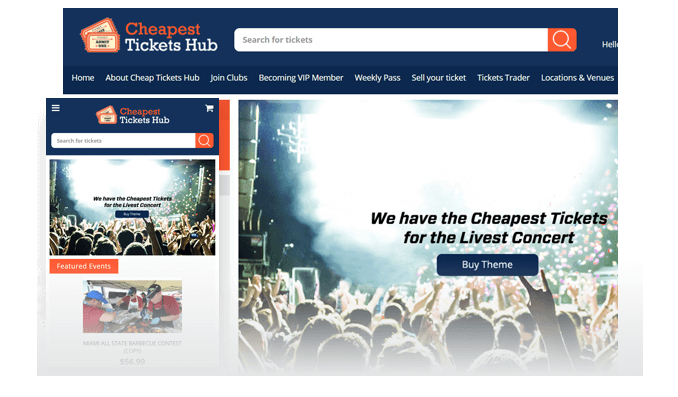The image appears to be a screen capture showcasing a website interface, likely for a ticket-purchasing platform. The screen is divided into two overlapping layers, each presenting a similar layout and theme.

**Layer 1: Primary Interface**
- **Header:** A navy background features the text "Cheapest Tickets Hub" in orange and white. Accompanying this header is an image of orange tickets with black font.
- **Search Box:** Below the header, a white search box with the placeholder text "Search for tickets" is prominently displayed. An orange box with a white magnifying glass icon is adjacent to it. To the right, "Hello" is written in white.
- **Navigation Menu:** 
  - "Home"
  - "About Cheap Tickets Hub"
  - "Join Clubs"
  - "Become a VIP Member"
  - "Weekly Pass"
  - "Sell Your Ticket"
  - "Tickets Trader"
  - "Locations & Venues"
- **Main Image:** A vibrant photograph of a concert with bright stage lights. Overlaid text in black reads, "We have the cheapest tickets for the livest concert." A blue and white button labeled "By Theme" is also present.

**Layer 2: Overlapping Interface**
- **Repeating Elements:** The layered image repeats several elements from the first layer, such as the navy header with "Cheapest Tickets Hub" in orange and white, the white search box, and the concert image with the blue and white "By Theme" button.
- **New Addition:** Below the repeated concert image, an orange and white box labeled "Featured Events" is included. There is a photograph of individuals dressed in red, wearing hats, and seemingly preparing food under a tent. Black font and a price are displayed underneath this photograph.

Overall, the image captures an overlapping, partial visualization of a ticketing website, highlighting key functionalities and showcasing concert and event details.